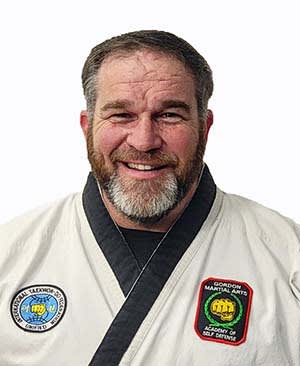This is a detailed photo of a man in his late 40s to early 50s, posed against a pure white backdrop. The image, captured from the chest up, showcases the man in a light beige Taekwondo gi accented with black trim along the lapels. Beneath the gi, he dons a black undershirt. The uniform features two distinct badges: on the left side, a circular emblem with a blue and yellow symbol surrounded by black text; on the right side, a black badge outlined in red with a white inscription and a yellow fist, reading "Gordon Martial Arts Academy of Self-Defense." The man sports a beard of gray and brown hues, matching his salt-and-pepper hair, which is close-cropped with gray streaking the sides. He is smiling broadly, revealing his top row of teeth, and his forehead has pronounced wrinkles, emphasizing his expression.